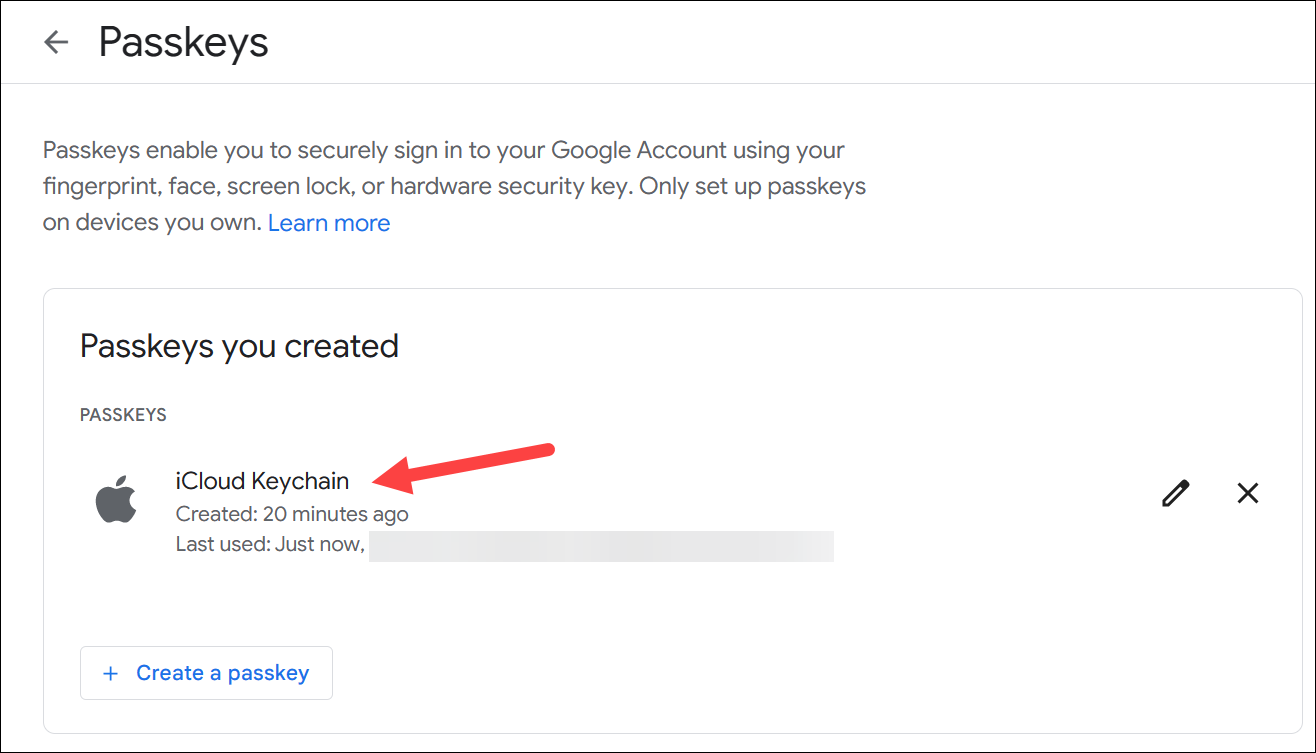**Caption:**

At the top of the image, there is a white rectangle featuring a left-pointing arrow and the words "Passkeys" written in bold black letters. Below this title, a paragraph explains that passkeys enable secure sign-in to your Google account using fingerprint, facial recognition, screen lock, or a hardware security key, emphasizing that passkeys should only be set up on personal devices. A blue hyperlink labeled "Learn more" follows the paragraph.

Underneath this section, another white rectangle is titled "Passkeys You Created." Listed beneath is the text "Passkeys," accompanied by the Apple logo with the inscription "iCloud Keychain" next to it. A red arrow points to the word "Keychain," indicating the passkey details: "Created 20 minutes ago" and "Last used just now."

On the far right, a filled gray rectangle contains a darker gray section with a pencil emblem and an X emblem toward the left. Beneath this, at the far left, there is another gray rectangle featuring a plus sign and the text "Create a passkey" in blue letters.